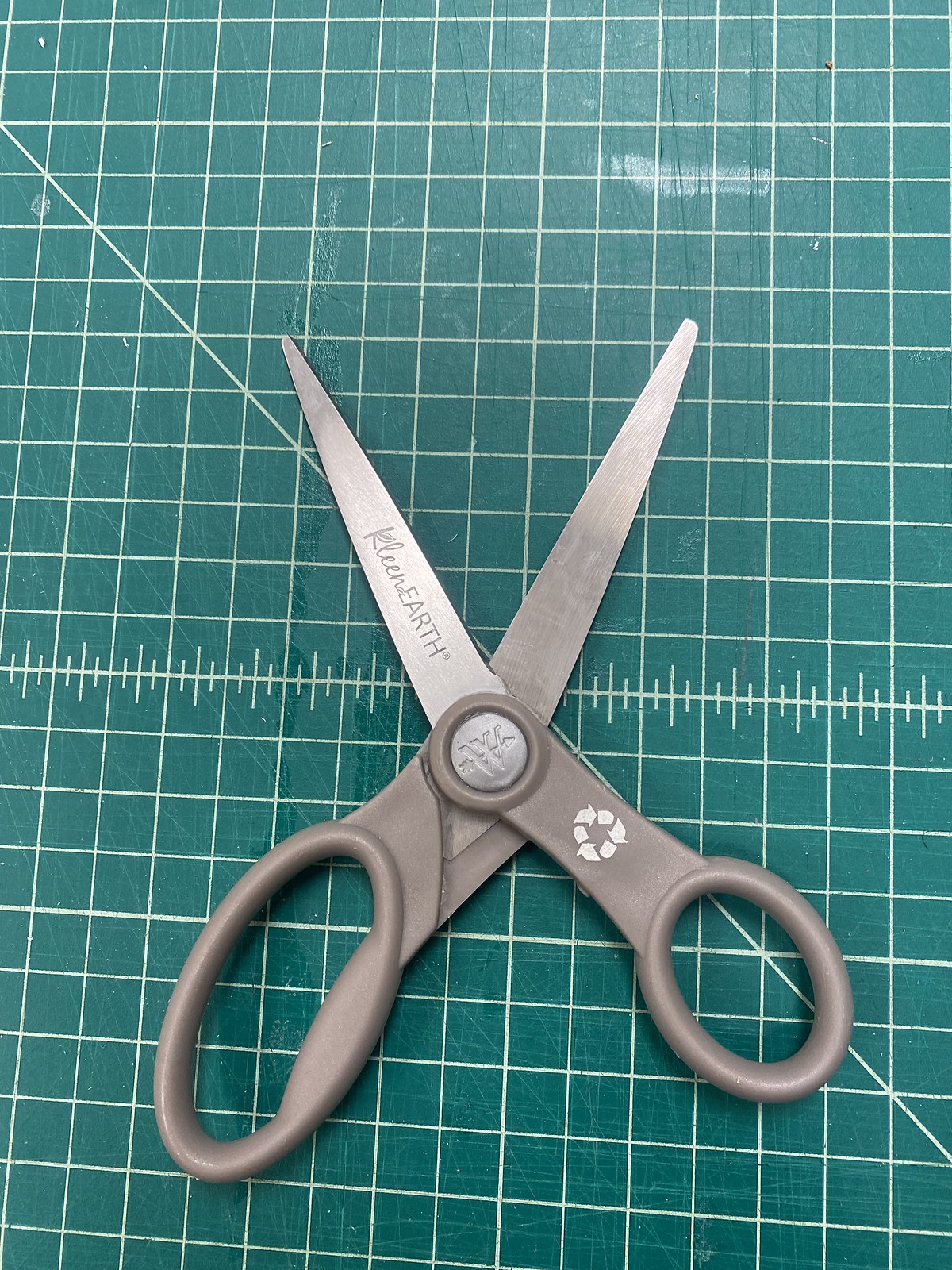This colour photograph showcases a pair of scissors with grey plastic handles and steely white blades. The scissors are open and facing upwards, with the larger finger hole on the left. Positioned atop a deep aqua surface marked by a white square grid pattern, the background resembles a sewing cutting mat. The mat features a diagonal white line from the top left to the bottom left and alternating vertical lines within the squares. A small white reflection is visible at the top. The right handle of the scissors displays a circular recycling logo. Written on one of the blades in script and print is the brand name: "KLEEN EARTH". Additional scaled markings on the mat include indicators like 1 1⁄2 and 1 1⁄4.